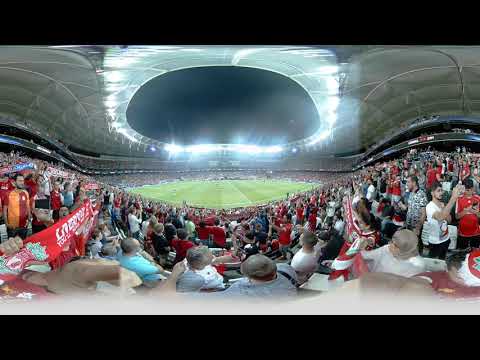This panoramic image captures the vibrant atmosphere of a football stadium. The stadium is densely packed with thousands of spectators seated across three-tiered bleachers, with some people standing, cheering, and interacting with one another. The green playing field at the center has an eye-like shape due to the panoramic effect, while the edges of the image are bordered by two black horizontal lines. The top part of the stadium features a curved structure adorned with numerous bright lights, creating a glowing ring around an open roof that reveals a clear, expansive sky. On the left side of the crowd, a fan can be seen holding up a red scarf with white letters, likely supporting Liverpool. The stadium itself has a modern, expansive design, emphasized by the 360-degree camera’s wavy, curved distortion that gives the image a dynamic, immersive quality.